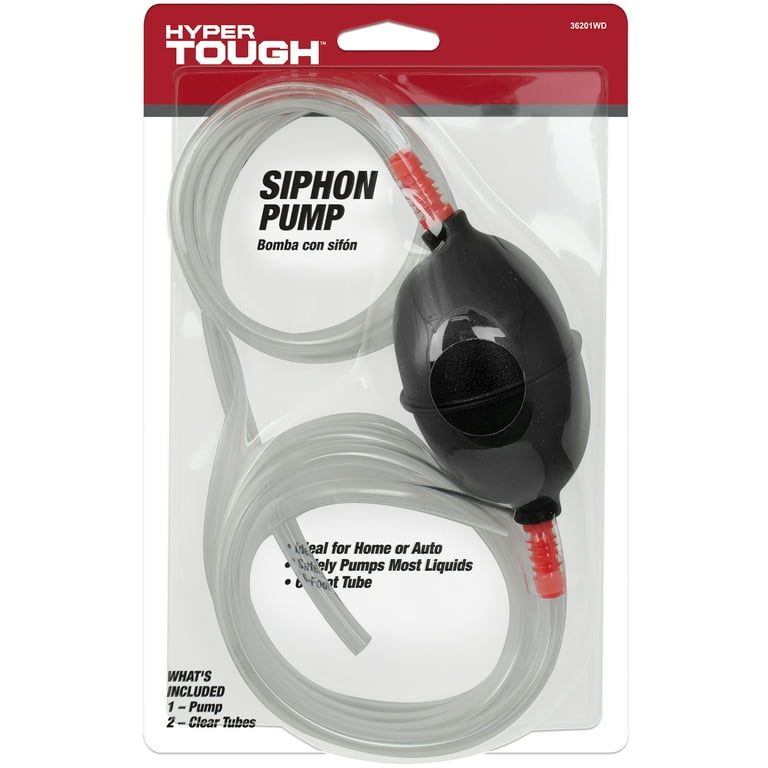This is a detailed product photo of the HyperTuff Siphon Pump, encased in its original packaging. The upper portion of the packaging features a red background with white lettering displaying "HYPER" in smaller font above "TOUGH" in larger font. This branding sits within a small band that comprises less than a third of the packaging’s total height. The rest of the packaging contrasts with a white background. Dominating the center, the product name "Siphon Pump" is prominently spelled out in large black letters, creating an outline of the coiled transparent tubing. The siphon pump includes a hand-compressible black rubber ball, engineered to create an airflow when squeezed, connected to the clear tubing via red corrugated fittings.

The transparent tubing winds into circular loops within the clear plastic casing, making it compact for packaging. Notably, the top circle showcases the words "Siphon Pump" in English, with the Spanish translation "Bomba Consilphone” underneath. The secondary circle contains additional descriptive text about the product, which is partially obscured by the tubing. In the bottom left corner of the packaging, "What's Included?" is clearly printed, with the specifics below it listing "1-Pump" and "2-Clear Tubes." The black pump ball is distinctly visible, accentuated by the red connectors that join it to the tubing. This siphon pump is designed for various uses, such as transferring gas from a tank or other liquid syphoning tasks for home or auto safety.